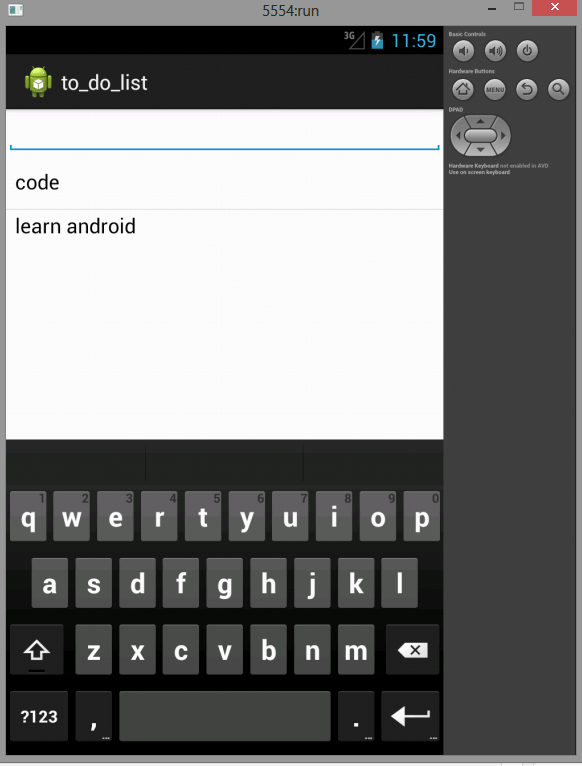The image showcases an app menu interface. The top section features a light gray bar, while the right side presents a dark gray column with several basic control buttons. These buttons include options to increase and decrease sound, and a power button to turn off the device. Below these, there are hardware buttons labeled "Home," "Menu," "Back," and "Search." Just beneath these controls is a directional pad for navigation, allowing up, down, left, or right movements.

Dominating the larger part of the image is a white background where a small robot icon is situated. Next to the robot, the words "To-Do List" are prominently displayed. Beneath this heading, two listed items are clearly visible: "Code" and "Learn Android."

Occupying the bottom third of the image is a virtual keyboard. This keyboard is set against a black background, with keys displayed in gray and white lettering for easy readability.